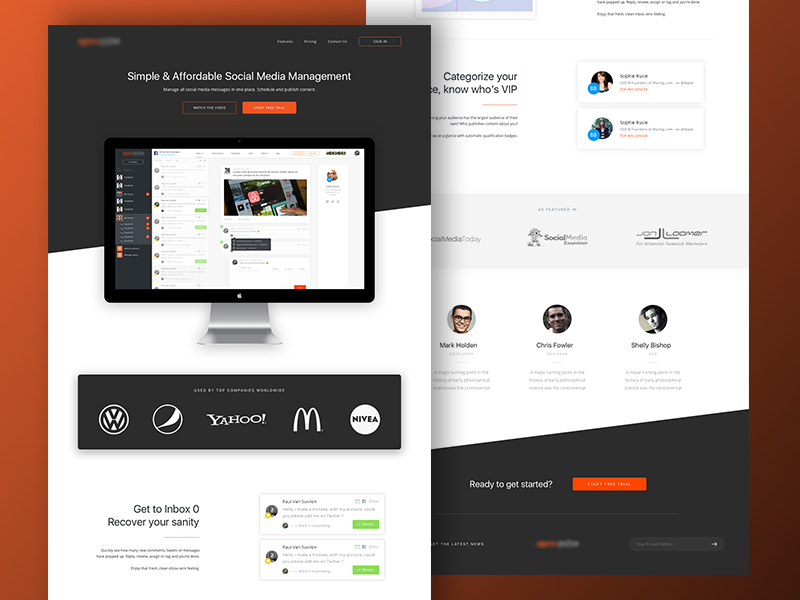In the image, there is an orange background with a slightly dark tone, overlaid by multiple pop-up windows. The primary pop-up is centered and divided into two sections: the top half is white and the bottom half is black. This pop-up prominently displays the text "Categorize your something, know your VIP" in black text. Additionally, this pop-up features various people’s profile pictures and some orange elements.

Overlapping this primary pop-up on the left side, another pop-up window appears. This secondary pop-up is also divided into sections: the top quarter is black while the remaining area is white. It contains the text "Simple and affordable social media management" alongside an image of a computer screen displaying indistinct content.

Below these sections, there is a band showcasing various well-known brand logos, including VW, Pepsi, Yahoo, McDonald's, and Nivea. Below this band, there's further text in black ink saying "Get in box zero, recover your sanity." The overall visual conveys themes of social media management and organization, highlighted by the blend of descriptive text and recognizable brand imagery.